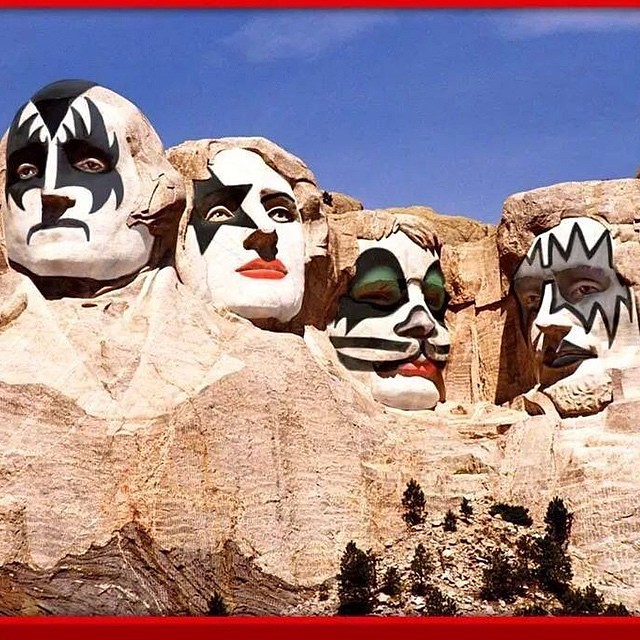This image appears to be an artistic parody or perhaps an AI-generated rendition inspired by the iconic Mount Rushmore Memorial. Instead of the traditional presidential faces, the artwork reimagines the figures with elaborate, gothic or clown-like makeup reminiscent of the band Kiss. Each of the four heads features distinct and theatrical modifications: 

- The first head, positioned where George Washington is typically located, has a white face with black lips and intricate black patterns, including a triangle extending down the forehead.
- The second head, replacing Thomas Jefferson, sports a white face with a black star over one eye and vibrant red lips.
- Theodore Roosevelt’s spot shows a character with a white face, black markings, and a greenish visor effect around the eyes, adding a unique twist.
- Lastly, the Abraham Lincoln figure is adorned with a silver and black visor-like design around the eyes, set against a white face.

The background features a clear blue sky with a minor wisp of cloud, enhancing the surreal and striking appearance of the transformed mountain range. Covering about 75% of the image from a quarter way down to the bottom, the scene also includes some trees at the base of the mountain and a red bar crossing the bottom with indistinct black marks or shadows.